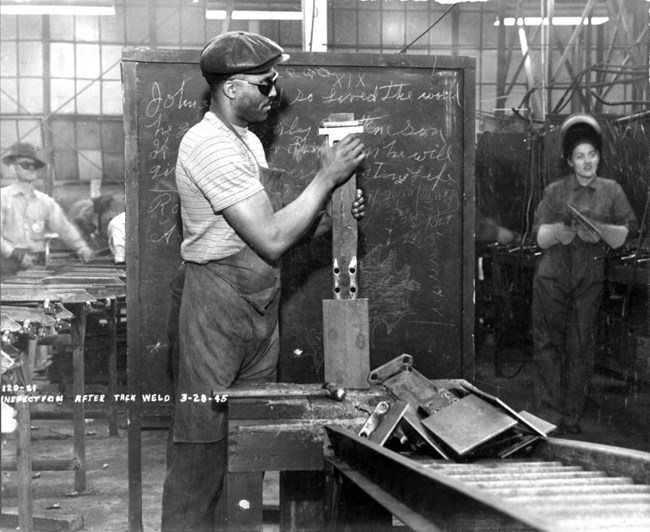This black and white photograph, likely from around 1945, captures a bustling industrial workshop. The central figure is an African-American man clad in a white striped t-shirt, apron, and a newspaper boy hat, complete with protective goggles. His hands grip a metal bar and a ruler, suggesting a task of careful measurement or inspection. Just behind him is a small blackboard with white chalk writing. Inscribed on it is a detailed notation, possibly reading "inspection after the weld 32845." Flanking him are other diligent workers; to the right, a woman in heavy-duty gloves and a welder's outfit is engaged in welding operations. Additional workers can be seen wearing goggles, hats, long-sleeved shirts, and gloves, busy at their respective stations. The workshop houses a conveyor belt laden with metal pieces, probably being transported for further processing. The background reveals more machinery, including metal parts with rivets, lights, and windows, reinforcing the setting of a bustling mid-20th-century factory or mill.